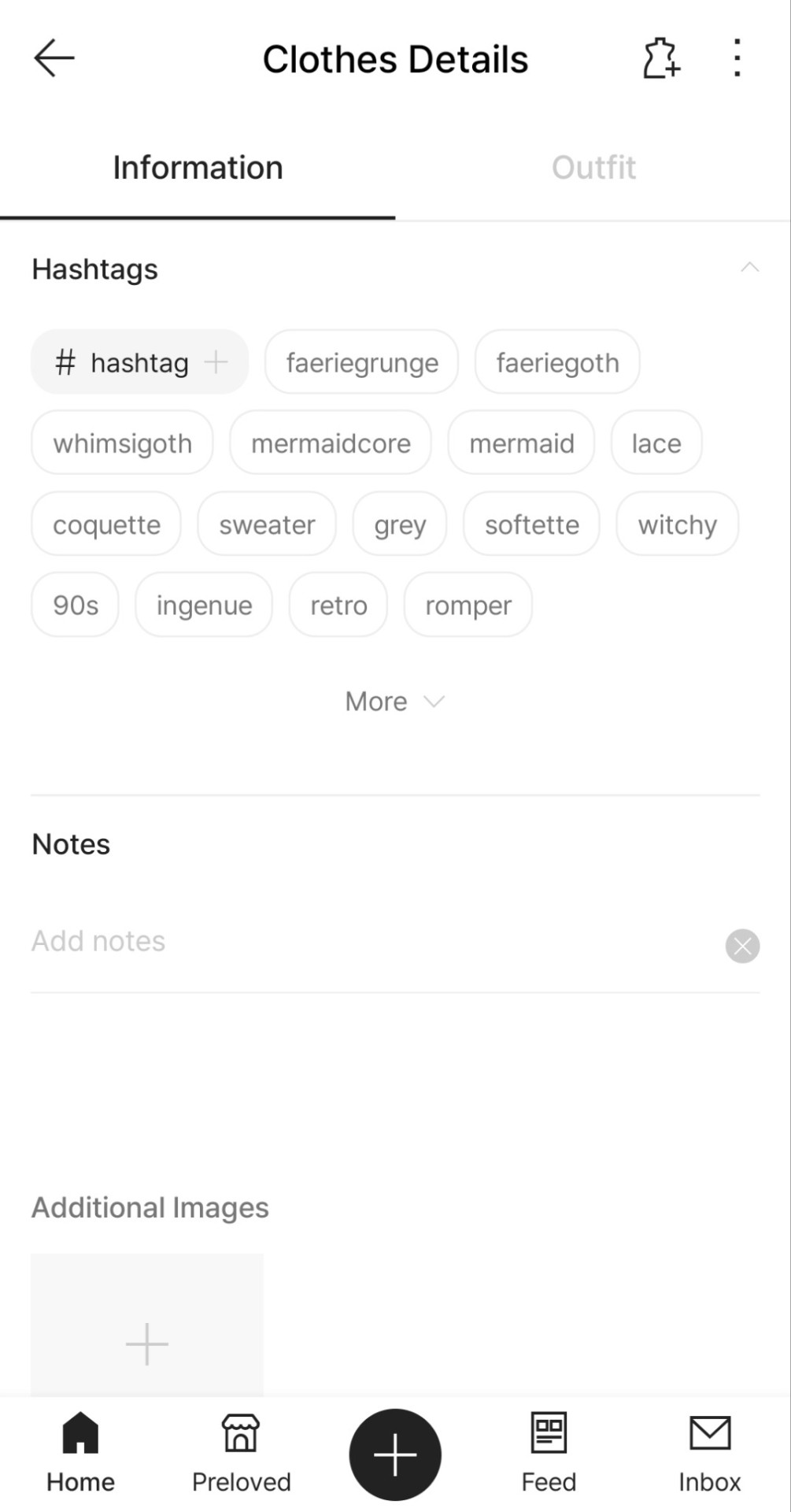In the top-left corner of the image, there is a small black arrow pointing to the left. Approximately three inches to the right, the title "Clothes Details" is prominently displayed at the top of the image. Towards the right side, there is an illustration of a mannequin outlined in black with a white fill. To the right of the mannequin is a small plus sign.

Beneath the mannequin image, the word "Information" is underlined, and adjacent to it is the word "Outfit". Below "Information", the word "Hashtags" is written, and next to it, inside a gray circle, there is a hashtag symbol followed by the word "Hashtag".

Moving further to the right, there are several categories listed. In the first row: "Fairy Grunge" and "Fairy Golf". In the second row: "Wim", "Wim", "Wims Golf", "Mermaid Core", "Mermaid Lace". In the third row: "Coquette", "Sweater", "Gray", "Soft At", "Witchy". In the final row: "90s Ingenuine", "Retro", and "Romper".

Below these categories, a long horizontal line spans the width of the image. Beneath this line, the word "Notes" is displayed, with an option to click and "Add Notes" underneath it. As you continue scrolling down, there is a section labeled "Additional Images" with a gray box featuring a plus symbol inside, indicating where additional images can be added.

At the very bottom of the image, starting from the left, there are several options: "Home", "Pre-Loved", a circle with a plus symbol inside, "Feed", and "Inbox".